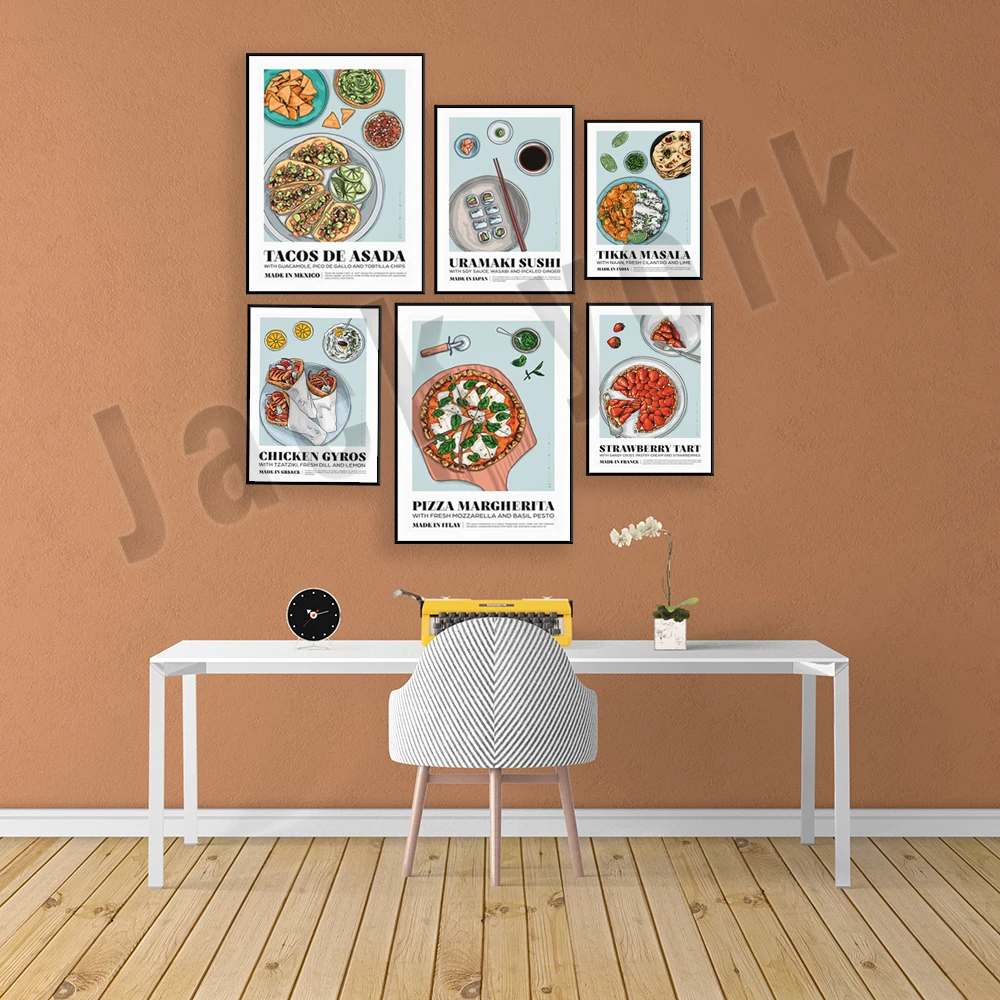The professionally staged and photographed, vertically rectangular image features a tasteful indoor scene under artificial lighting. The setting is an office space against a medium brown wall, complemented by a light brown wooden tile floor and a white baseboard at the bottom. Centered against the wall is a sleek, white table with a white, cushioned chair that has three wooden legs. The table is adorned with three distinct objects: a small round alarm clock on the left corner, a vibrant yellow typewriter with black keys in the center, and a yellow square planter with white flowers on the right. Arranged above the table are six vertically rectangular artistic illustrations of various foods, including tacos, pizza, chicken, and shish kebab, adding a dynamic visual interest. The image has a diagonal watermark across it that reads "Jack York" in big block letters.